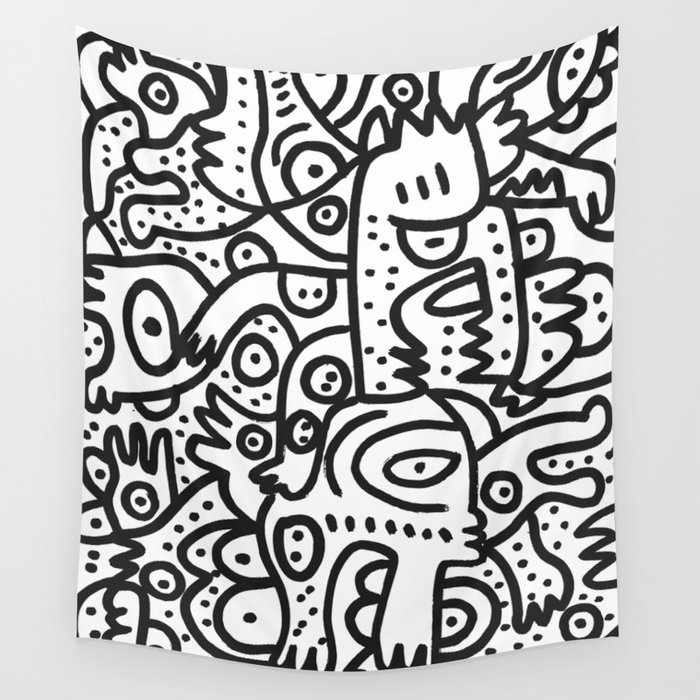This image features a black and white line art style drawing mounted on an off-white light gray wall. The artwork, displayed on a slightly curved fabric tapestry, predominantly fills the frame, allowing only a small border of the wall to be visible. Reminiscent of Keith Herring's style, the piece showcases thick black lines forming semi-abstract shapes of faces, bodies, animals, and people, with an abundance of dot work. The drawing, which looks as though it was created with a very fat black marker, contains numerous face-like objects and eye-like circles with dots, interspersed with squiggles and hand-like forms with three curves resembling fingers or feet. The minimalistic, shadow-free line work invites viewers to interpret the shapes, perceiving different figures and forms hidden within the intricate design.